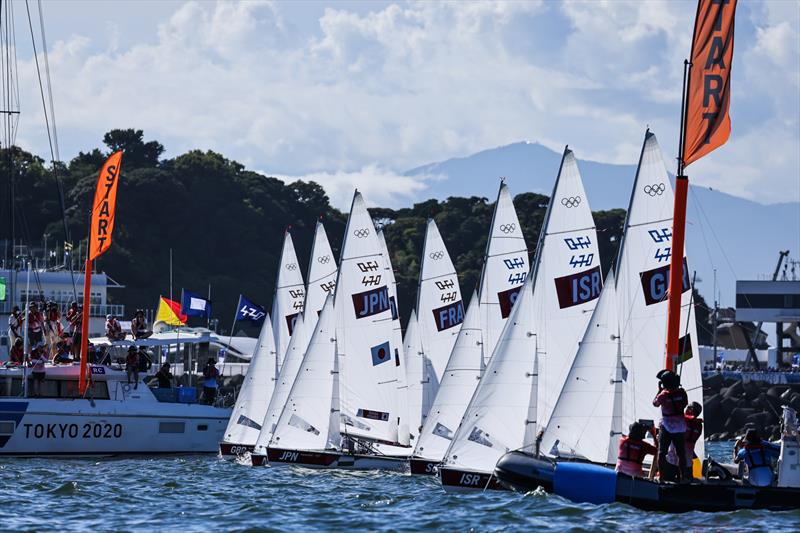This captivating photograph captures the thrilling commencement of a sailing regatta. Eight small sailboats are impeccably lined up at the starting line, poised and ready to race. To the right of the assembled boats, a larger vessel is anchored, prominently displaying a mast with a flag that reads "START." On the opposite side, another boat similarly bears a "START" flag, signaling the official beginning of the race. Notably, the boat on the far side features the inscription "Tokyo 2020," indicating that this competitive event is taking place in Tokyo. The serene background is graced with the lush greenery of trees, the majestic rise of mountain ranges, and a picturesque sky adorned with scattered clouds. The photograph effortlessly captures the palpable excitement and scenic beauty of the moment.